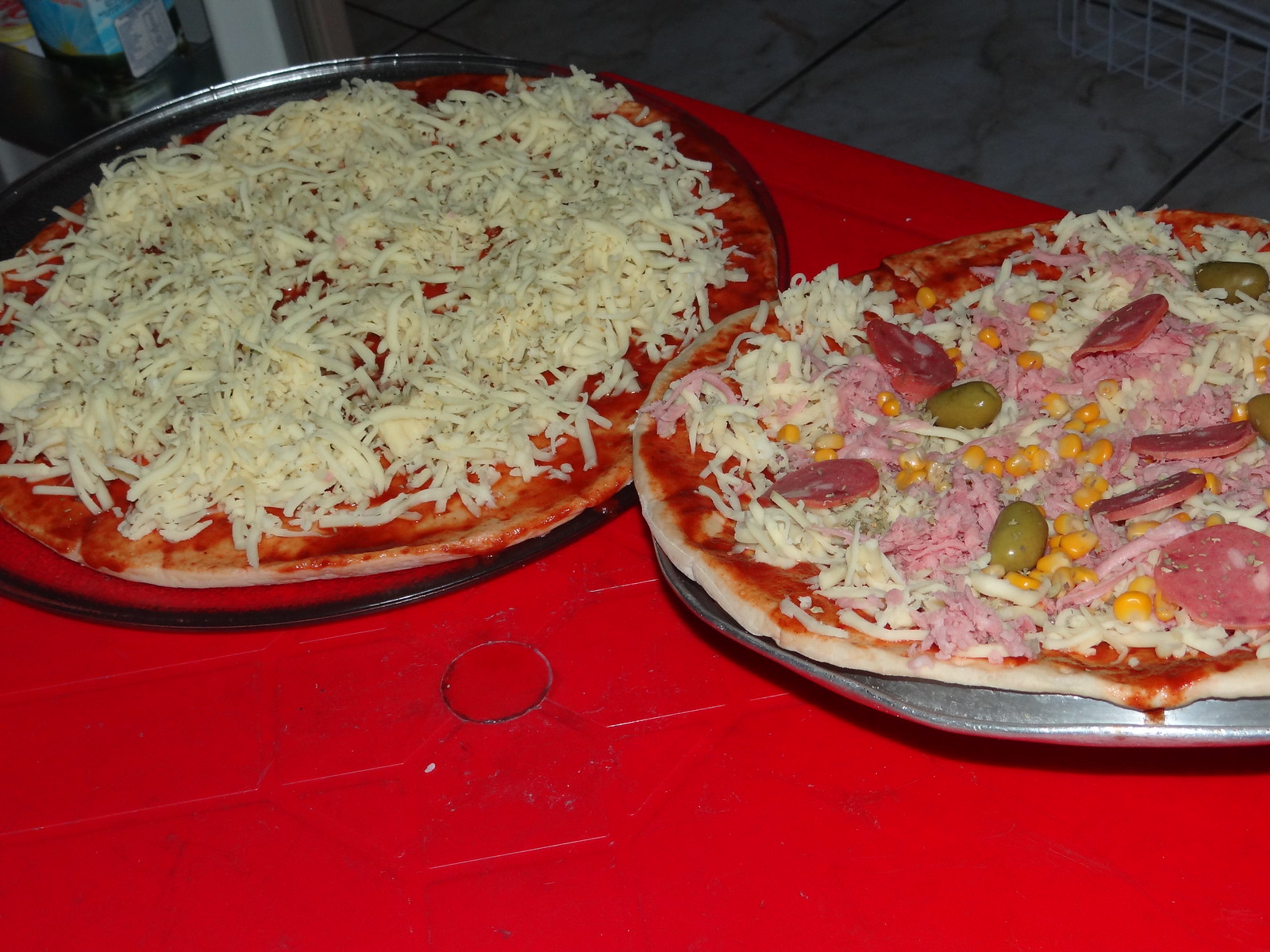The photograph shows two unbaked pizzas sitting on metal baking pans placed on a red tablecloth. The pizza on the left features a generous amount of mozzarella cheese over a tomato sauce base, creating a classic all-cheese pizza ready for the oven. The right pizza, which might be considered less conventional to some, is topped with dried tomatoes, salami, ground bologna or spam, green olives, and corn, along with the usual sauce and cheese. Both pizzas are situated on a marble tile floor, and part of a tea bottle is just visible in the upper left corner near the cheese pizza.